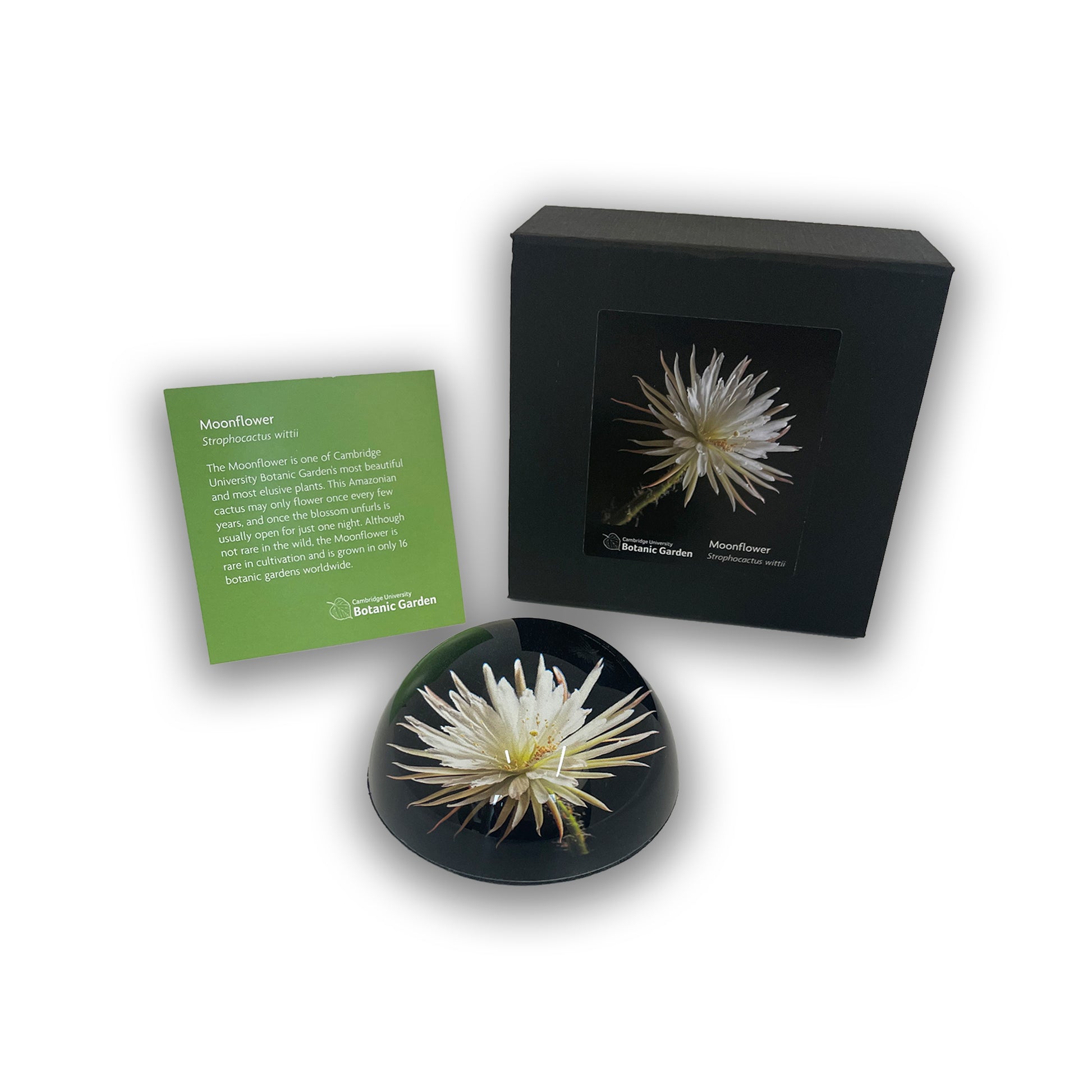The image displays a product showcase with a clean white background. Featured prominently is the Moonflower (Strophocactus wittii), heralded as one of Cambridge University Botanic Garden's most beautiful and elusive plants. The display includes a green booklet on the left-hand side that provides detailed information about the Moonflower, noting its rare blooming cycle, where the American cactus may only flower every few years and typically unfolds its blossom for just one night.

Adjacent to the booklet is a black box featuring a photo of the Moonflower. Centrally positioned at the bottom of the image is an actual Moonflower encased in a glass globe, reminiscent of a snow globe, providing a clear view of the delicate blossom. This detailed and informative display artfully combines visual and textual elements to highlight the rarity and beauty of the Moonflower.